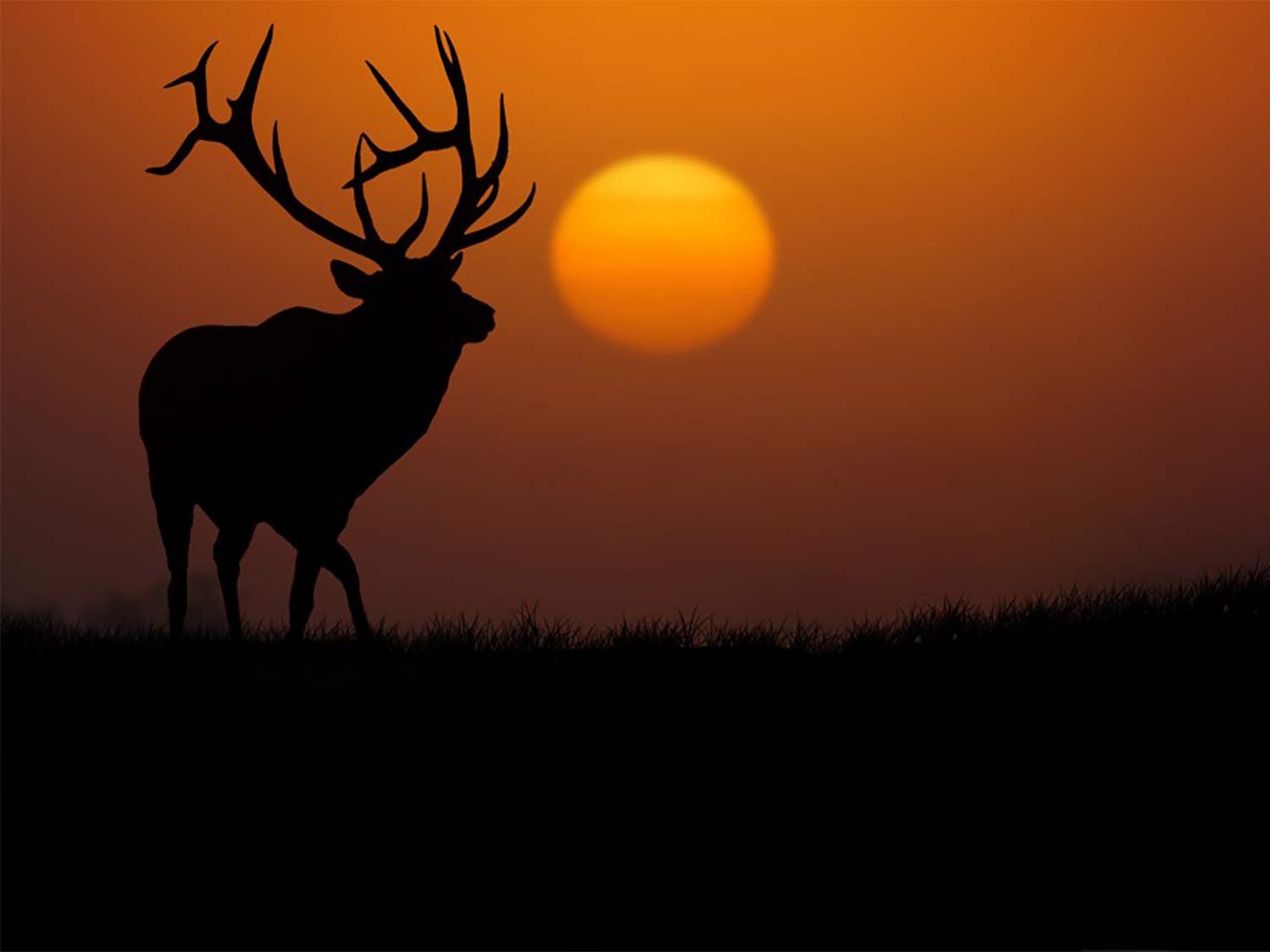The image captures a stunning silhouette of a large male elk, prominently featuring its impressive, sharp antlers. The elk stands in a field of tall, dark grass, facing left but seemingly turning to walk towards the right side of the image. The scene is bathed in the ambient glow of a setting sun, which appears as a radiant, hazy orb of deep orange and yellow hues, gradually blending into the dark auburn and grayish tones of the sky. The contrasting lighting creates an evocative outline of the elk and the grassy field, adding depth and drama to the landscape. Near the center left of the image, the faint silhouette of a tree further accentuates the serene and majestic atmosphere of this twilight moment.